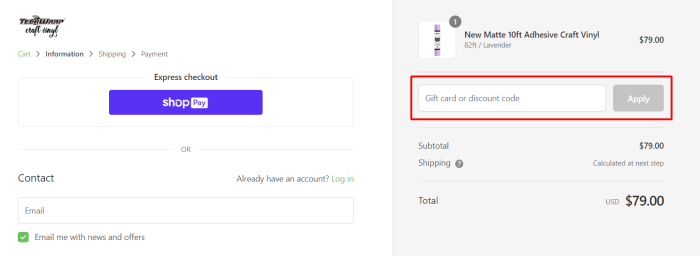This composite image comprises two distinct sections, each presenting different elements of an online shopping process. 

On the left side, set against a white background, there is a small, somewhat difficult-to-read logo situated in the upper left corner. The logo appears to spell "TWOW," followed by smaller, less legible text beneath it. Directly below the logo, a breadcrumb navigation bar is presented: the word "CART" is in gray font with a small black arrow pointing right next to it, followed by the word "INFORMATION" in black font with another right-pointing black arrow adjacent to it. Continuing in gray font are the words "SHIPPING" and "PAYMENT," each separated by small right-pointing black arrows. 

Below the breadcrumb navigation, in prominent black font, the words "EXPRESS CHECKOUT" are displayed. There is a blue rectangle beneath this text containing the text "SHOP PAY" in white font. Below this button, the word "OR" is written in gray font, followed by the text "CONTACT," also in black font. Further below is the phrase "I already have an account" and the word "LOGIN" highlighted in yellow font. The bottom section features a field for entering an email address, supplemented by a small orange checkbox labeled "EMAIL ME WITH NEWS AND OFFERS."

On the right side of the composite, a gray rectangle stands out. In the top left corner of this section, there is a white square showcasing an image of what appears to be a tube of paint. Directly to the left of this image, there is a description written in black font: "NEW MAT 10-FOOT ADHESIVE CRAFT VINYL," followed by the price, "$79."